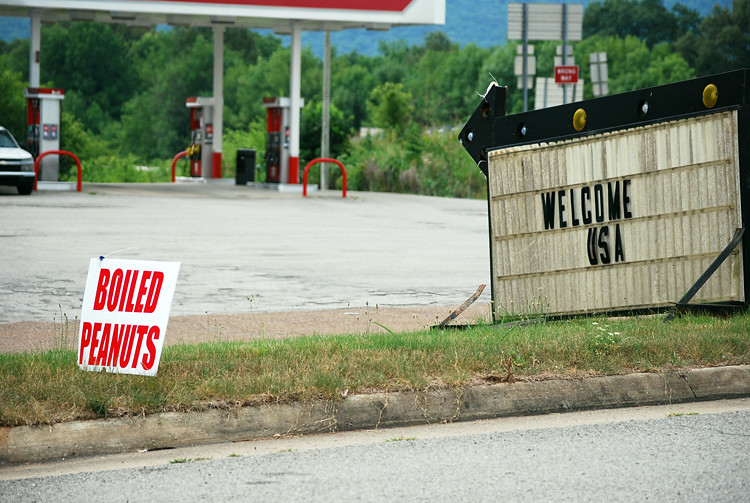The photograph captures a roadside sign prominently displayed on a small patch of grass. The main sign, white with bold black text, reads "Welcome USA" and features an arrow at the top pointing to the left. In front of this, another smaller sign advertises "Boiled Peanuts" in red text against a white background. Behind these signs, a gas station with a red and white color scheme is visible. On the left side of the image, a white truck partially appears, presumably as its owner refuels at the station.